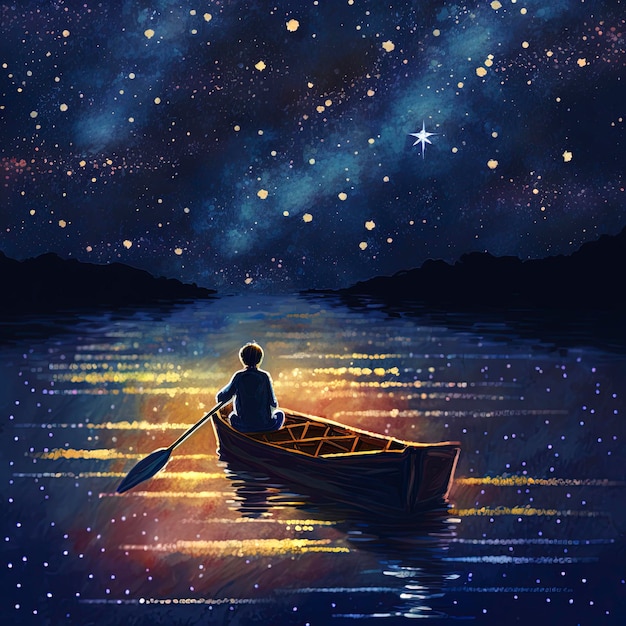This detailed and surrealistic illustration depicts a young boy with short hair sitting towards the front of a canoe, holding a paddle in his left hand against the backdrop of a calm, serene lake under a nighttime sky. The boy’s back faces the viewer, adding a sense of solitude and mystery to the scene. The night sky is a rich, dark blue, sprinkled with numerous small, twinkling yellow stars and dominated by one large, white North Star. The stars' reflections create a mesmerizing display of bright yellow and orange hues on the tranquil water's surface, adding a magical aura to the image. In the distance, silhouettes of mountains rise against the sky. The scene is further enhanced by surrealistic elements, such as the path of the boat being outlined with horizontal striations in gold and yellow, adding an ethereal quality. This illustration, seemingly created by an adult, possesses the charm and wonder perfect for a children's book, yet it could equally be admired as a piece of art in a gallery.